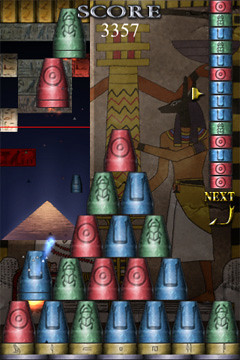This detailed screenshot from a video game depicts a vibrant Egyptian-themed scene. The top of the image features the word "SCORE" in gray letters, with a score of "3357" displayed in white numbers beneath it. The background showcases intricate Egyptian-style paintings, highlighting the god Anubis with his distinctive jackal head, looking to the left. A pyramid structure is also visible in the left background. The foreground presents an array of colorful, inverted cups stacked in a pyramid formation. The cups vary in color—red, blue, and green—and each color features a unique design: a red cup with a circle, a blue cup with a U-shape, and a green cup with a scarab beetle. On the right side of the screen, there is a vertical stack of thick rings, mirroring the colors and designs of the cups. Beneath this stack, "NEXT" is written in gold letters. The overall image suggests a cup-stacking game set within an Egyptian motif.